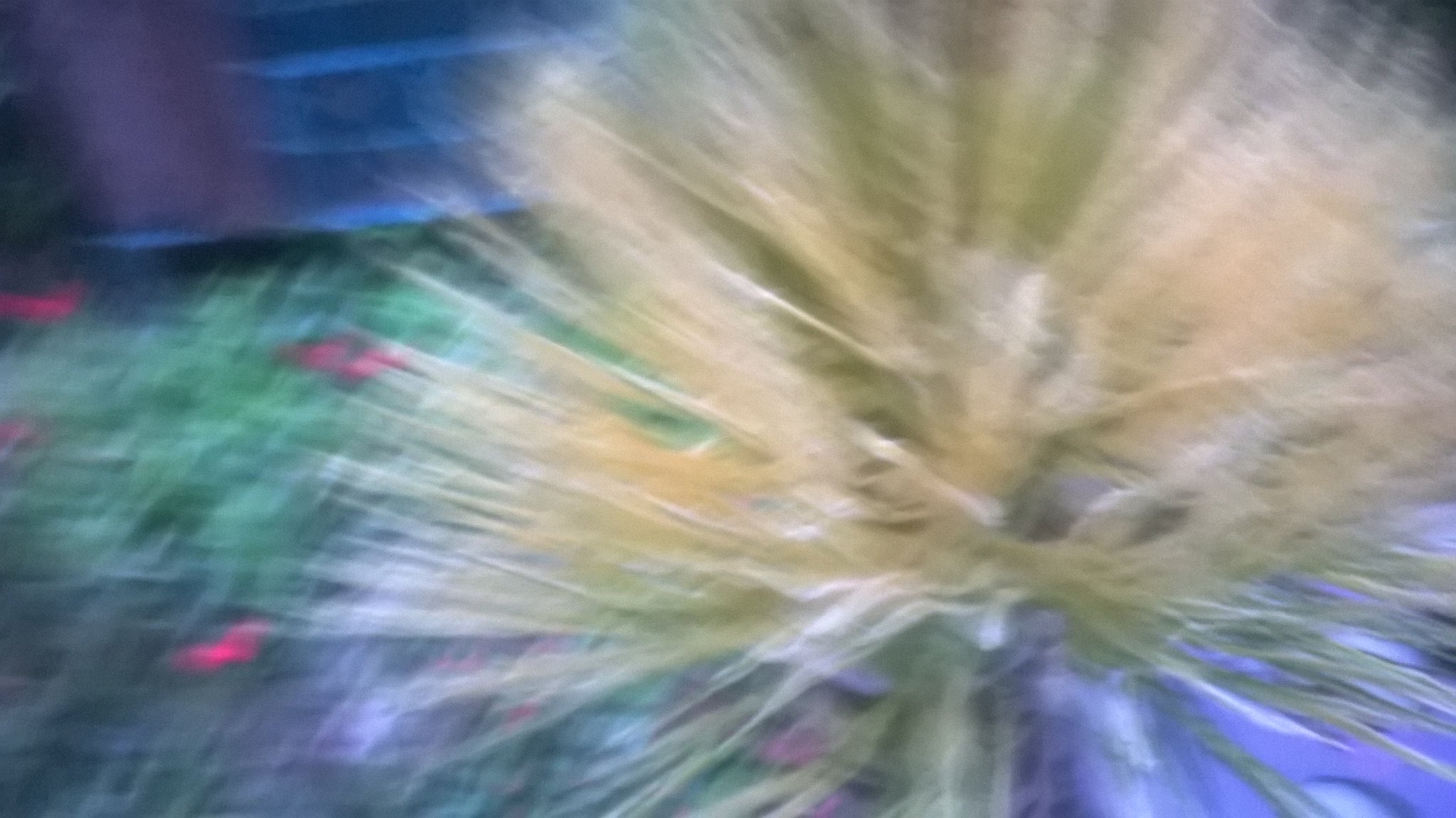The image is a very blurry photograph, seemingly taken outdoors in a first-person perspective, possibly while in motion. Dominating the right half of the image is a tall, fluffy grass bush or palm-like plant with wheat-colored grass emerging from its center and fanning out. The plant features both brown and green hues. On the left side, more green shrubbery can be seen in front of what appears to be a building with a red brick wall. This building has a mixed structure that may include a white section or a protruding brick, making it ambiguous. Hints of bluish-purple color appear to the right, although their exact nature is indistinct due to blur. The scene appears to be captured at dusk, emphasizing the dark and moody ambiance.